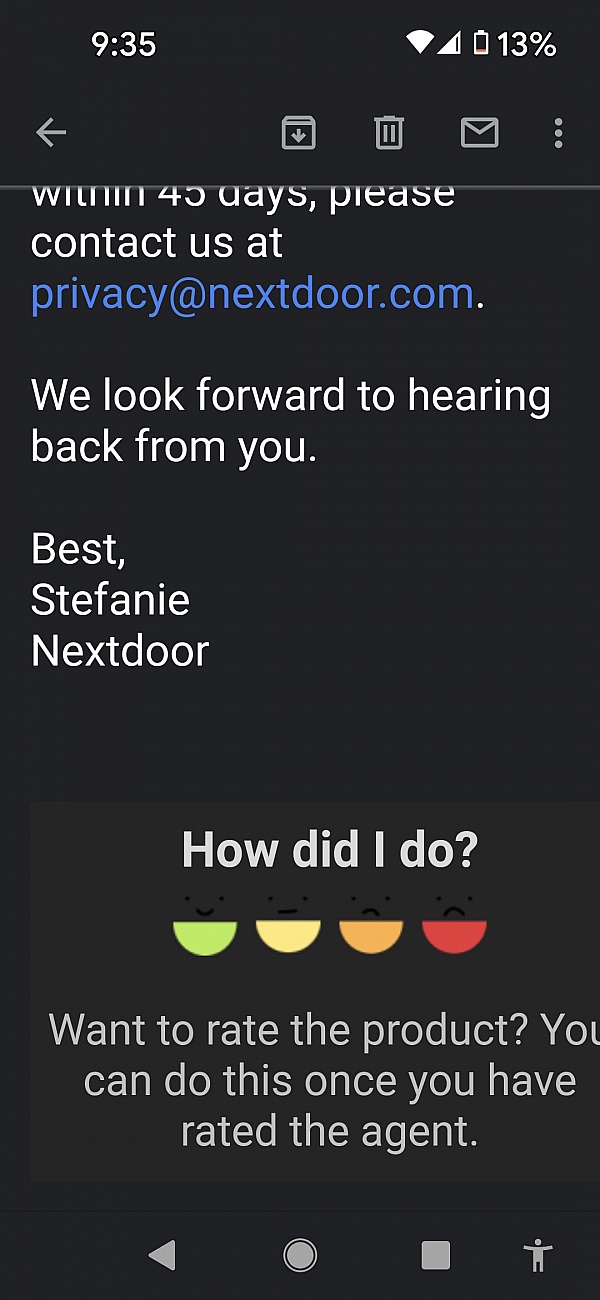**Detailed Caption:**

The screenshot displays a smartphone interface with a predominantly black background. The status bar at the top of the screen shows it is 9:35 AM, with a strong signal and a low battery level of 13%. Below the status bar, various icons are present, including a left-pointing arrow, a trash can symbol, an envelope, and three vertical dots.

Prominently featured in the middle section of the screen is a message in two colors: the contact request "Within 45 days, please contact us at" is highlighted in blue, followed by the email address "privacyatnextdoor.com" in white. Additionally, a follow-up sentence reads, "We look forward to hearing back from you. Best, Stephanie Nextdoor."

The lower portion of the screen appears to be segmented, providing a feedback section titled "How did I do?" which is accompanied by four half-circle rating options, each with a different color: lime green, peach, salmon, and orange. Below this is an instruction that reads, "Want to rate the product? You can do this once you have rated the agent."

At the very bottom of the screen are navigation buttons including a back button, a home button, a person icon, and a close button.

This detailed layout effectively guides the user through the feedback process while providing essential contact information.